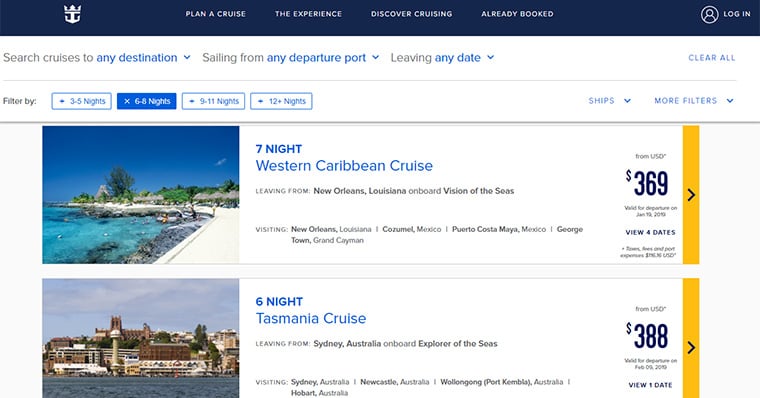This image is a screenshot taken from a computer, showcasing a cruise booking website under the brand "Planet Cruise." The website features a horizontal layout typical of computer screens. At the top of the webpage, there are navigation options including "The Experience," "Discover Cruising," and "Already Booked," alongside a login option. Users can search cruises based on various criteria such as destination, departure port, departure date, and trip duration. The duration filters available are 3-5 nights, 6-8 nights, 9-11 nights, and 12+ nights. 

In the screenshot, the 6-8 night filter is selected, displaying two highlighted cruises. The first offering is a 7-night Western Caribbean cruise departing from New Orleans aboard the "Vision of the Seas." The itinerary includes stops at New Orleans, Mexico, Puerto Costa Maya, and George Town in Grand Cayman, with prices starting at $369. The second option is a 6-night Tasmania cruise from Sydney, Australia on the "Explorer of the Seas," visiting Sydney, Newcastle, Wollongong, and Hobart. 

The page is a comprehensive hub for planning cruise vacations, allowing users to tailor their trips to specific preferences easily.